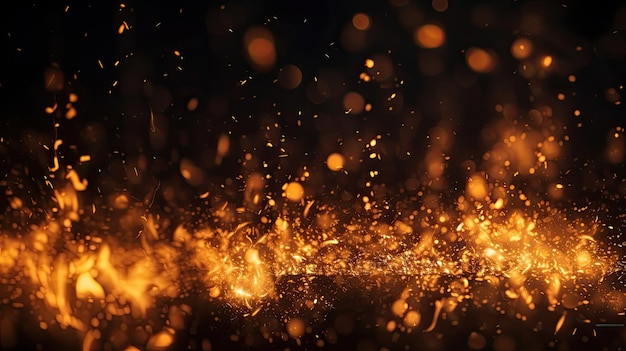The image depicts a close-up view of glowing embers and sparks, creating a mesmerizing and dynamic scene of fire. The fiery display stretches in a horizontal line across the photograph, with vibrant, dancing flames that are lush with hues of orange and red. These flames and embers rise into a stark black sky, illuminated beautifully against the dark background. The scene is both eerie and warm, as the amber glow bathes the darkness in a vibrant, almost celebratory light. Flecks of embers, resembling both sparks and droplets, ascend into the air, adding a sense of movement and lightness to the scene. The simplicity of the black, orange, and yellow color scheme makes the imagery pop, generating a striking visual contrast. Despite the abstract nature of the image, its atmospheric quality evokes the raw energy and beauty of a fire glowing intensely in the night.